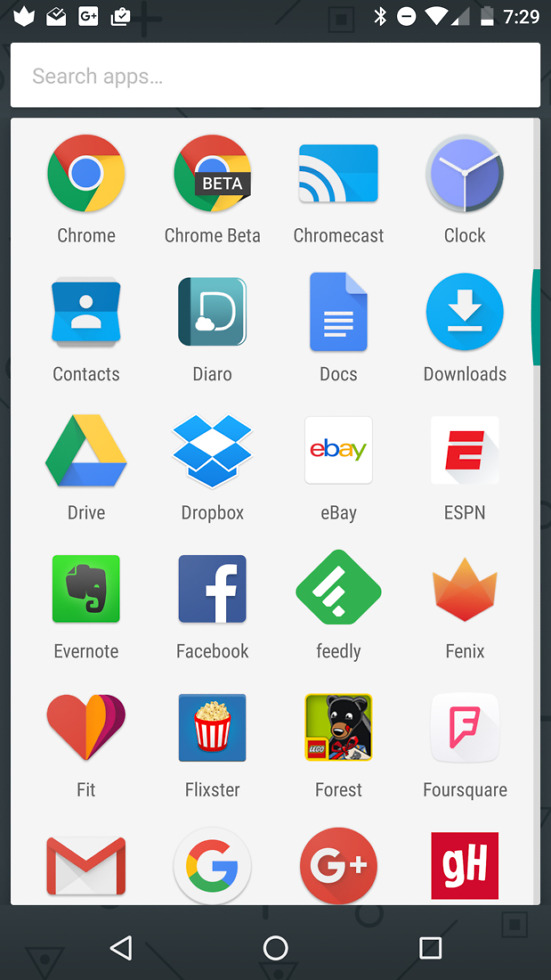The image displays the screen of a tablet, which appears wider than a typical smartphone. Arranged neatly are the application icons, distributed across four columns and six rows. The topmost row includes Google Chrome, Chrome Beta, Chromecast, and Clock. The subsequent rows feature the following icons:

- **Second row:** Contacts, Diario, Docs, Downloads.
- **Third row:** Drive, Dropbox, eBay, ESPN.
- **Fourth row:** Evernote, Facebook, Feedly, Phoenix.
- **Fifth row:** Fit, Flixster, Forest, Foursquare.
- **Sixth row:** Gmail, Google, Google+, GH.

At the very top, there is a search bar spanning the width of the screen. The notification bar displays several icons: a white symbol resembling a leaf, an envelope, a Google+ icon, a square, and a suitcase with a check mark. Additionally, status indicators reveal that Bluetooth is on, Do Not Disturb mode is active, the device has a full Wi-Fi connection, a partial data signal, and low battery. The time shown is 7:29.